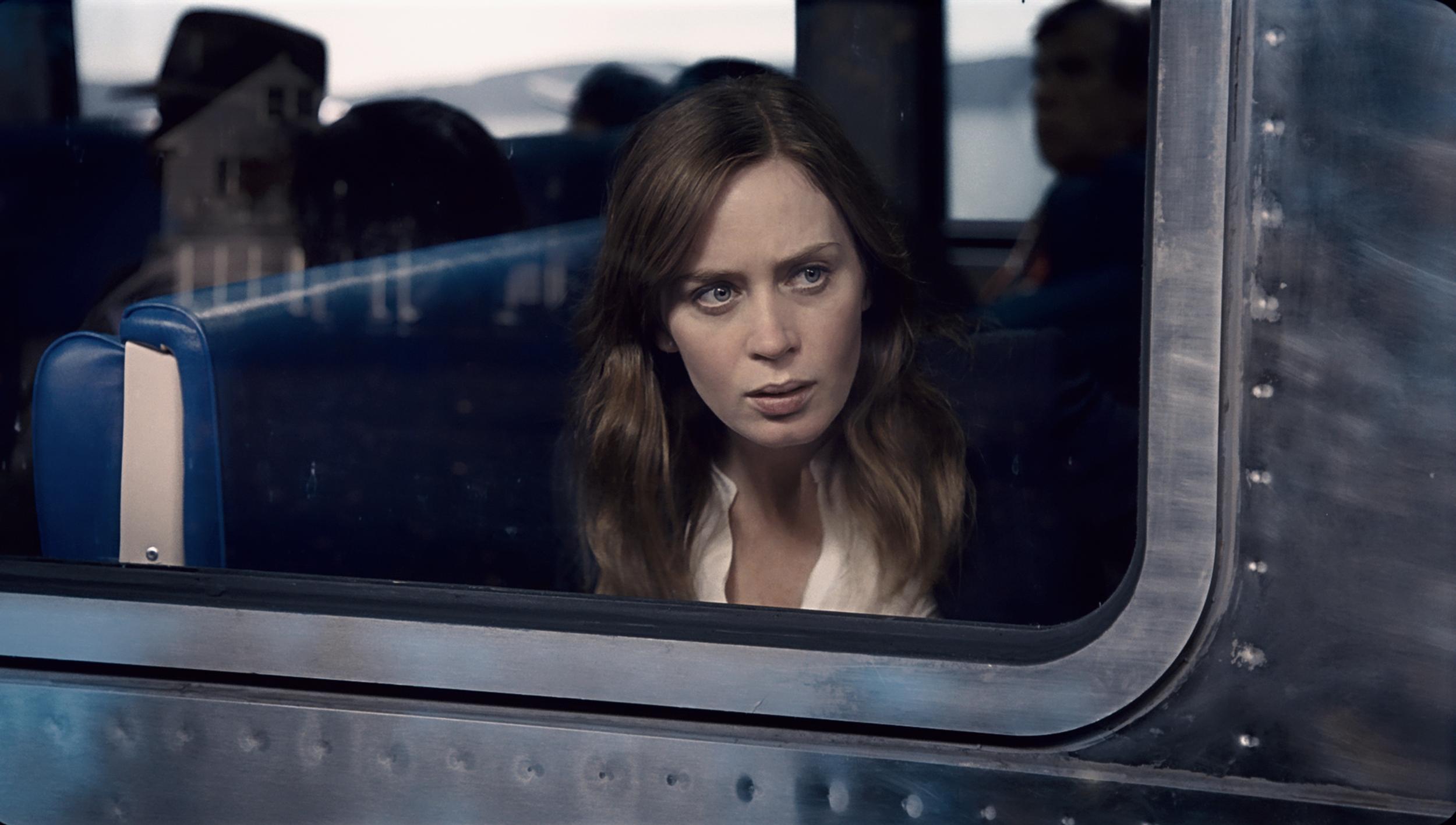This detailed image captures actress Emily Blunt, known for her role in "The Girl on the Train," as she sits in a blue seat of a metal train, peering pensively out the window. The scene is zoomed in, making the setting ambiguous if not for her known affiliation with the film. Emily's brown hair frames her solemn face, her gray eyes reflecting a mix of concern and contemplation as she gazes outside. She's wearing a cream-colored shirt, though the rest of her attire is obscured in shadows. Behind her, the blurry silhouettes of several other passengers, including a distinguishable man's hat, fade into the background. The window beside her offers a vague reflection of a house and possibly some distant water or hills, adding layers of ambiguity to her troubled expression. The external view of the train highlights its shiny, studded metal exterior, further emphasizing the confinement and introspective mood of the scene.